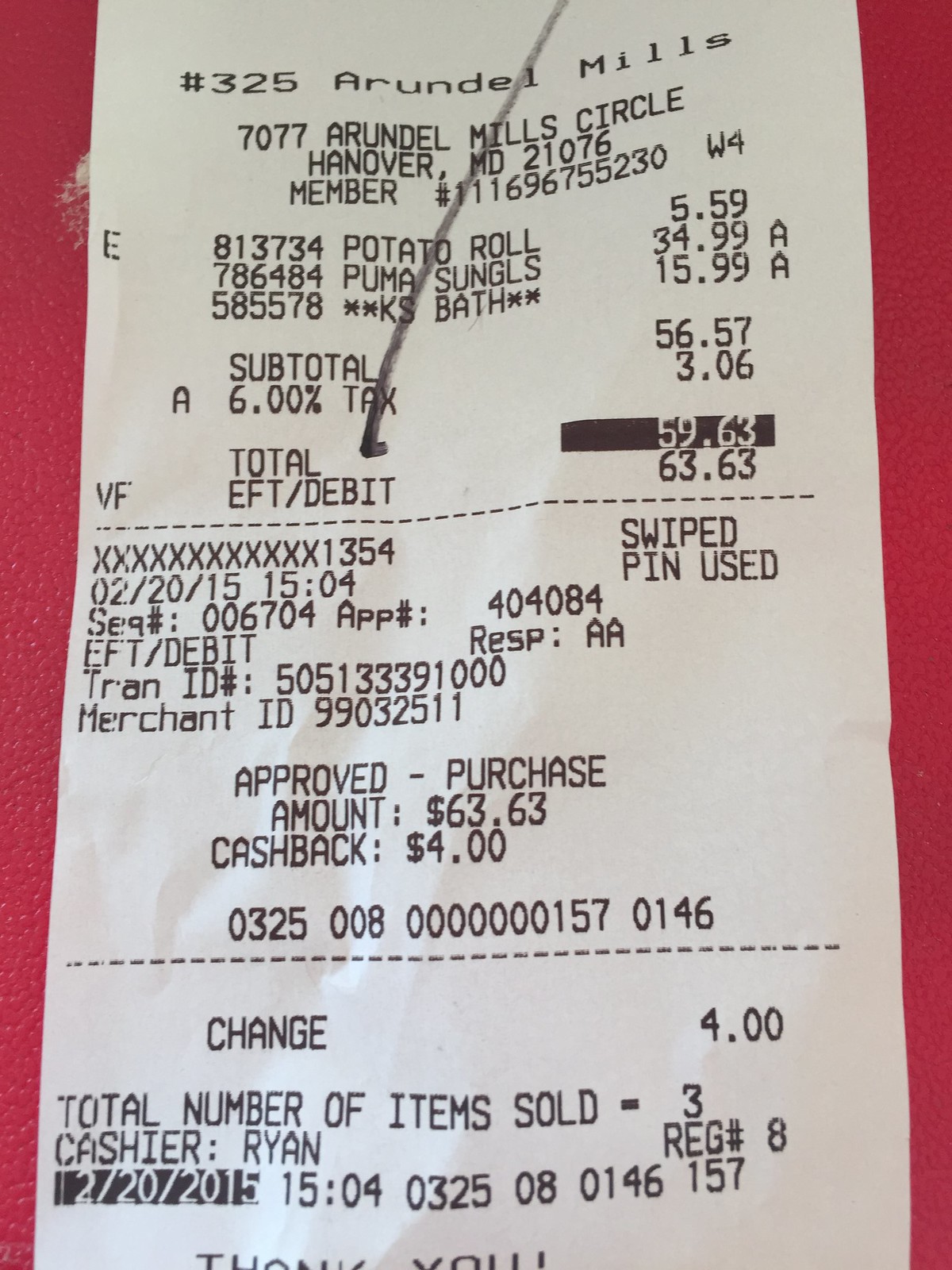This is a detailed, close-up photograph of a white receipt with black printing, laying on a dark pink, almost red leather or embossed vinyl surface. The receipt runs vertically, and a thin red border frames the left and right sides where it meets the background. Across the top, slightly right of center, a black mark made with a marker slashes diagonally downward to the left approximately one-third of the way down the receipt. 

At the top, in bold black letters, it reads "Arundel Mills #325," followed by the address "7077 Arundel Mills Circle, Hanover, Maryland 21076." The receipt lists the following purchased items: a potato roll for $5.59, Puma sunglasses for $34.99, and a KS bath item for $15.99. The subtotal stands at $56.57 with an additional 6% tax amounting to $3.06. This makes the total $59.63.

The payment details show that a debit card was used, displaying the last four digits of the card number, with the notation that the card was swiped and a PIN was used. The total payment approved was $63.63, including $4 cash back, resulting in change of $4. The receipt also includes the purchase date, cashier number, and total number of items sold, which is three.